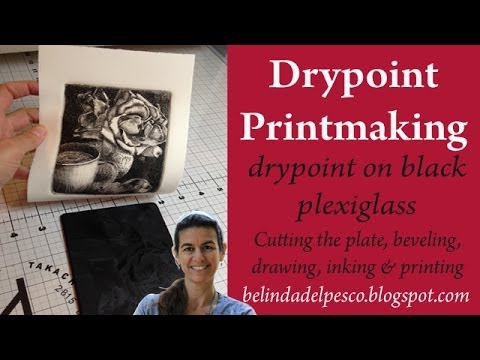The image is an advertisement for drypoint printmaking, featuring a black stripe at the top and bottom. On the left side, there’s a photo illustrating a drypoint chart used for cutting prints for framing. A hand is holding up a black-and-white photo intended for framing. The right side contains text detailing the printmaking process: "Drypoint on black plexiglass, cutting the plate, beveling, drawing, inking, and printing," and includes the URL belindadelpesco.blogspot.com.

In front of the chart stands a woman with black hair draped over her shoulder, tilting her head slightly. She is dressed in a green shirt and is holding the photo above a unique notebook. The precise execution of the drypoint technique and the careful step-by-step illustration make this advertisement informative for those interested in printmaking.